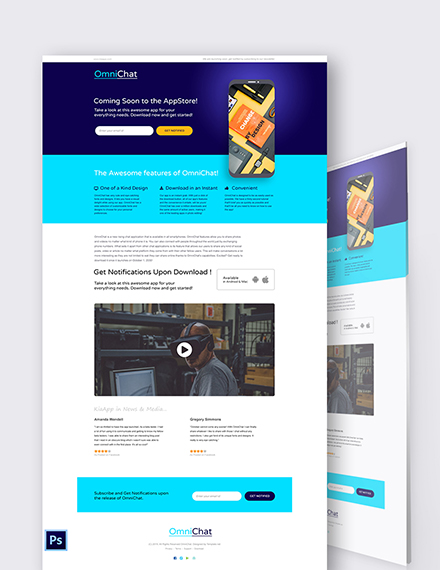The image appears to be a screenshot of an online advertisement for an upcoming app called OmniChat. Dominating the top-left corner of the image is the OmniChat logo, accompanied by the text "Coming soon to the App Store." Below this is a paragraph of text, though it's too blurred to decipher. Adjacent to the paragraph is a search bar and a prominent yellow action button, the function of which is not specified. 

On the right side of the image is a superimposed graphic of a smartphone, illustrating a visual of the app. The upper part of the page features a dark blue stripe with the headline "The awesome features of OmniChat," under which three headers are listed, each accompanied by a short, unreadable paragraph of text. 

The main section of the page has a white background and includes a lengthy paragraph at the top that begins with "Get notifications upon download." Centrally located is a video showcasing a person wearing a VR headset.

A lighter blue stripe crosses the lower part of the background, but it does not extend the full width of the image. This blue stripe contains another search bar and an additional action button. Between this stripe and the central video, there are two user reviews, each accompanied by star ratings, though the text is too small to read.

To the right of the main content, there appears to be another page displayed at an angle, resembling a smaller version of the primary page but with illegible text.